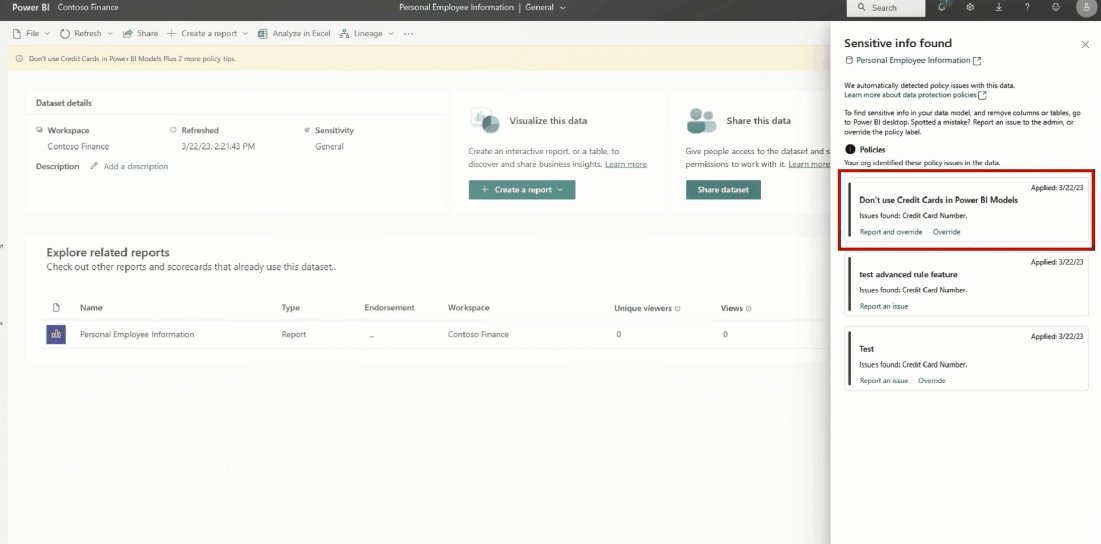This screenshot appears to be from a computer, specifically showcasing a software interface that closely resembles Power BI, with a reference to "Contosa Finance." At the top-left corner, the words "Power BI" and "Contosa Finance" are prominently displayed. The central section of the screen is titled "Personal Employee Information," followed by a subheading "General" with an associated drop-down menu.

Directly below, a menu bar lists options such as File, Refresh, Share, Create a Report, Analyze in Excel, and Lineage. Beneath this, detailed information about the data set is presented, including the Workspace labeled "Contosa Finance," the most recent refresh date of March 22, 2023, and a sensitivity classification labeled as General.

On the far right side of the interface, there are options to visualize the data, presumably enabling the creation of graphs or charts, and to share the data set. An informative section advises users to "Explore Related Reports," indicating that other reports and scorecards utilizing this specific data set already exist.

A highlighted message on the right side of the screen warns about sensitive information, stating "Sensitive Info Found. Don't use credit cards in Power BI models." This ensures users are cautious about the type of data included in the Power BI models.